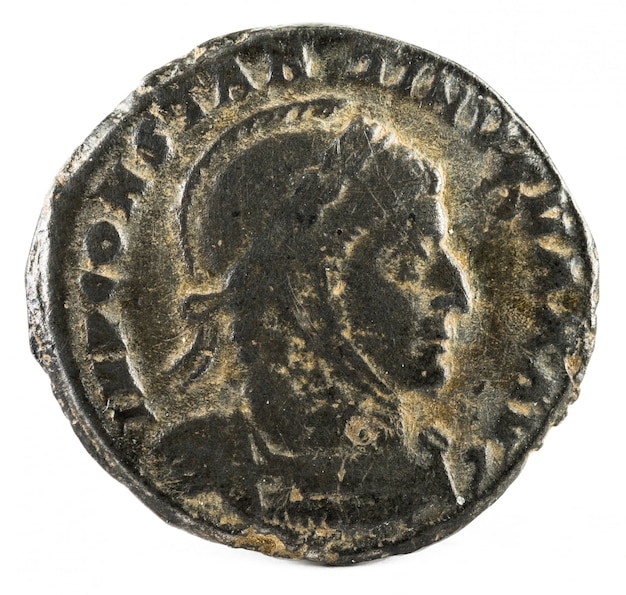This image depicts a worn, ancient coin that appears to originate from the Greek or Roman period. The coin is an imperfect circle, displaying a dark gray or black coloration with hints of yellow or beige patina. Central to the coin's design is the profile of a man with a pronounced nose and a serious, neutral expression, looking to the right. His head is adorned with what seems to be a helmet, characteristic of Greek iconography. Encircling the upper edge of the coin are weathered inscriptions in a non-English script, with some letters resembling 'S', 'N', 'T', and 'A', though they are difficult to discern due to the coin's age and condition.